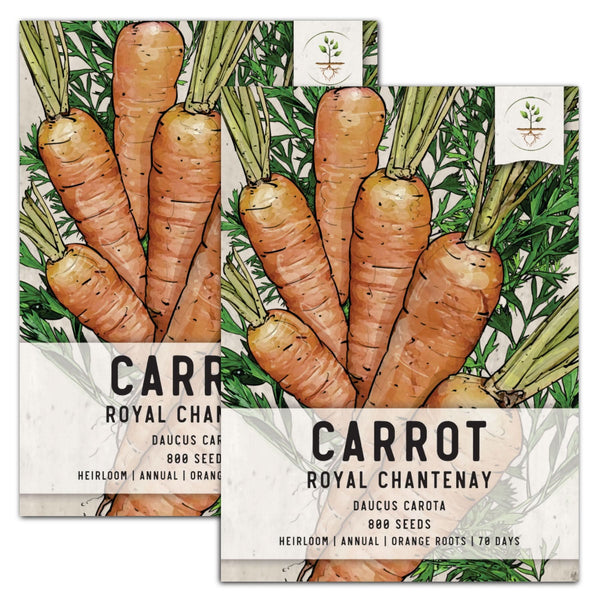The image depicts two identical rectangular packets of Royal Chantenay carrot seeds, displayed against a solid white background with one packet slightly overlaid on the other. Each packet features an illustrated bunch of six orange carrots with thick green leaves sprouting from the tops, set against a backdrop of green foliage. The packaging includes a white banner at the top right showing an illustration of a plant with roots. At the bottom of each packet, a white rectangle contains text that reads, "Carrot, Royal Chantenay, Dacus carota, 800 seeds, heirloom, annual, orange roots, 70 days." This detailed packaging suggests the seeds are suitable for someone aiming to plant and grow a substantial number of heirloom Royal Chantenay carrots.